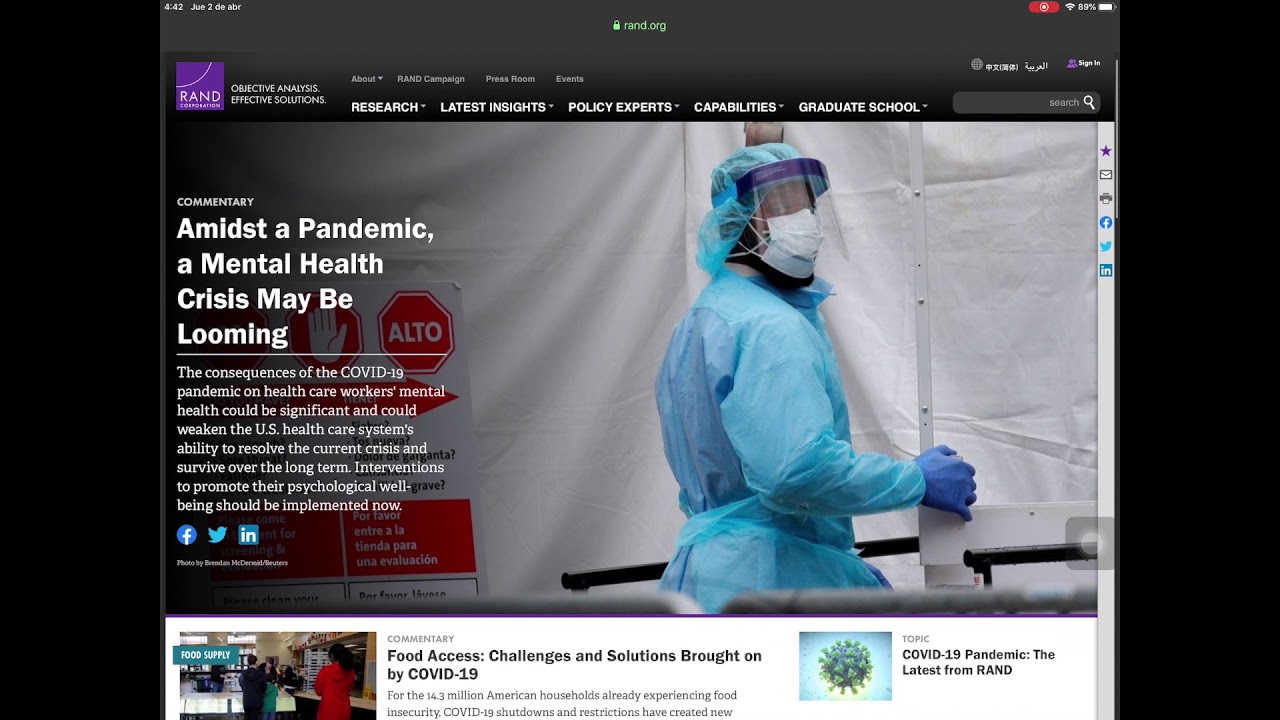The image is a screenshot of the ran.org webpage taken at 4:42 PM on June 2nd. The top of the image shows several status icons: a red button, a Wi-Fi icon with a percentage, and a battery icon. Directly underneath, the URL "ran.org" is displayed in green with a lock icon preceding it, indicating a secure connection.

The header of the webpage features the RAND logo alongside their slogan, "Objective Analysis. Effective Solutions." Below the header, a navigation menu includes buttons labeled "About," "RAND Cover Page," "Press Release," and another icon that appears to represent "Email or Events."

Further down, a secondary menu with larger buttons offers links to sections such as "Research," "Latest Insights," "Policy Experts," "Capabilities," and "Graduate School." A search bar is situated below this menu.

The main content of the page highlights a commentary titled "Amidst a Pandemic and Mental Health Crisis May Be Looming." Accompanying the text, there is an image of a person wearing protective gear, which includes a blue face mask, a face shield, and a white heavy-duty mask.